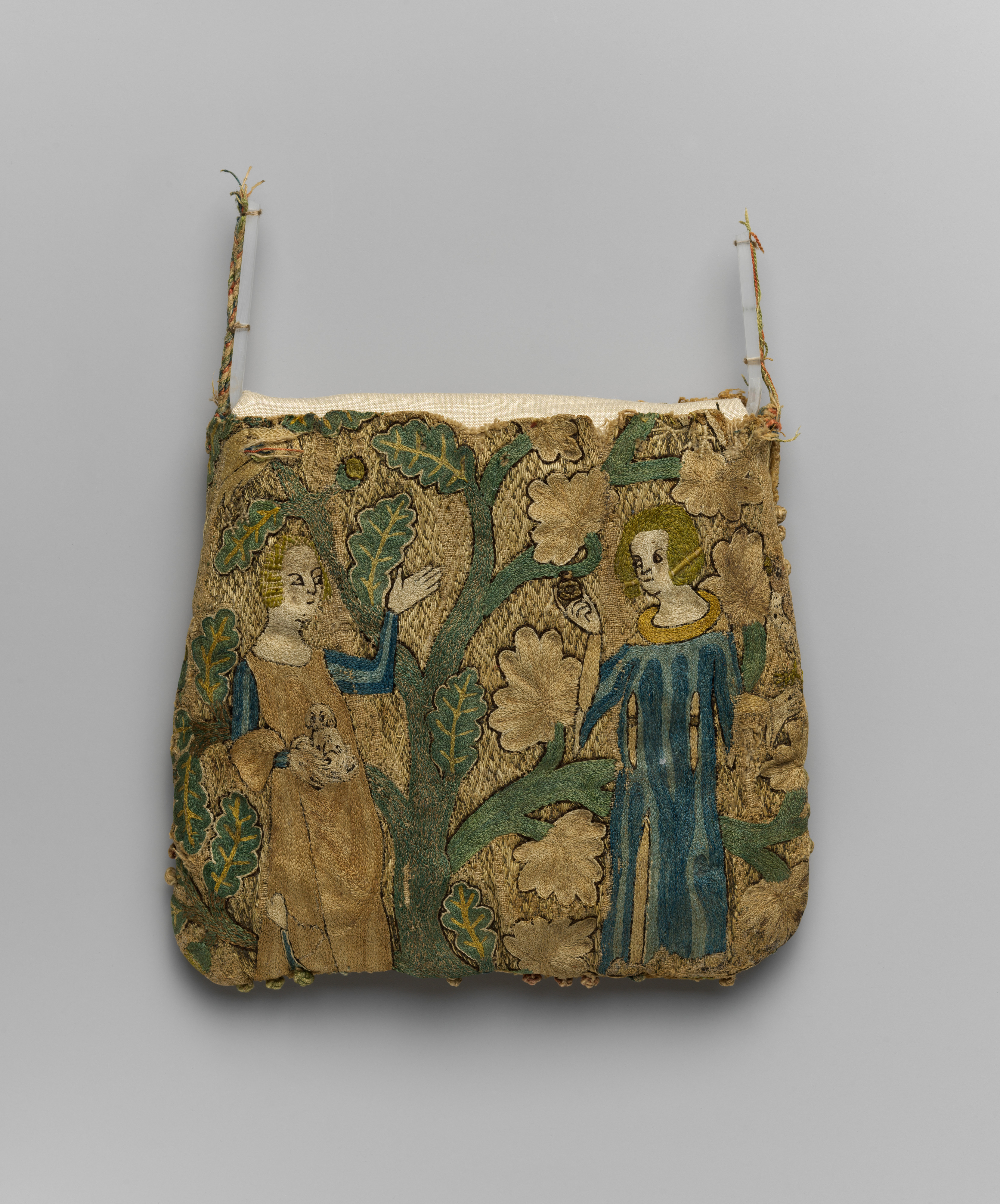The image shows a vintage, hand-embroidered satchel bag set against a light gray background. The bag has a square shape and features a delicate gold and blue hand-embroidered scene. The embroidery depicts two women in elegant, 18th-century style gowns, standing on either side of a large, central tree with detailed green and yellow-brown leaves.

On the left, a woman with blond hair is dressed in a long tan dress with puffy sleeves. She has her right hand raised and appears to be holding an image, possibly of an animal. On the right, a second woman with goldish hair wears a blue gown that has visible slits and a gold collar. She is seen touching a piece of fruit hanging from the tree. Both women have intricate details in their robes, with shades of blue and gold. 

The tree between them is detailed with veins in the leaves and extending branches. The satchel shows signs of distress, suggesting its age and handmade origin. It is suspended by two short, rope-like handles on either side, lending it a vintage charm.